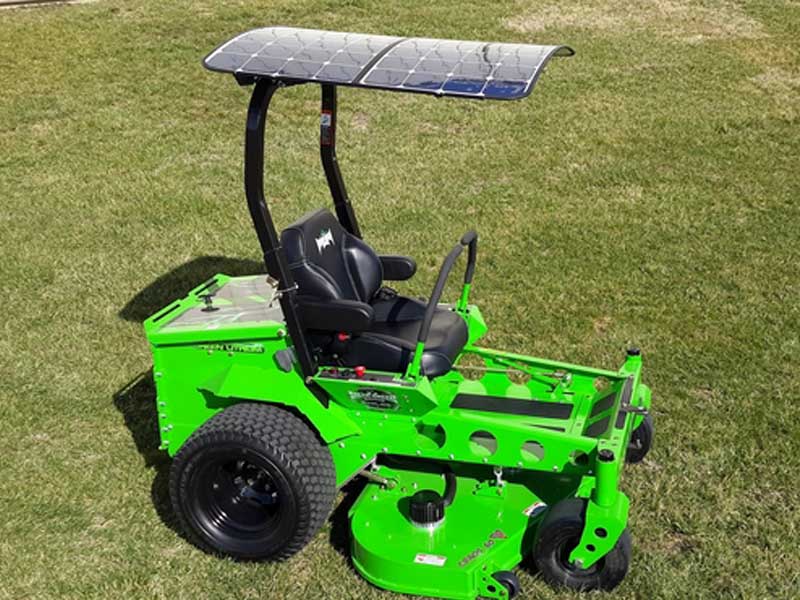A vivid, neon green lawnmower, potentially commercial-grade but suitable for personal use, sits prominently on a well-trimmed, sunlit lawn of mixed green, yellow, and brown hues. The lawnmower features a black, leather-upholstered seat with armrests, enhancing driver comfort. Overhead, a structural frame supports a brown-gray roof equipped with solar panels, providing shade and sustainable power. The machine is built using visible I-beams with perforations and has four wheels: smaller, dark front tires that resemble casters, and larger black-rimmed back tires. Control is managed via two levers that flank the seat, enabling precise maneuverability. Additional white, gray, and red accents are visible, and although the text on the machine is unreadable, the overall design is both functional and striking.